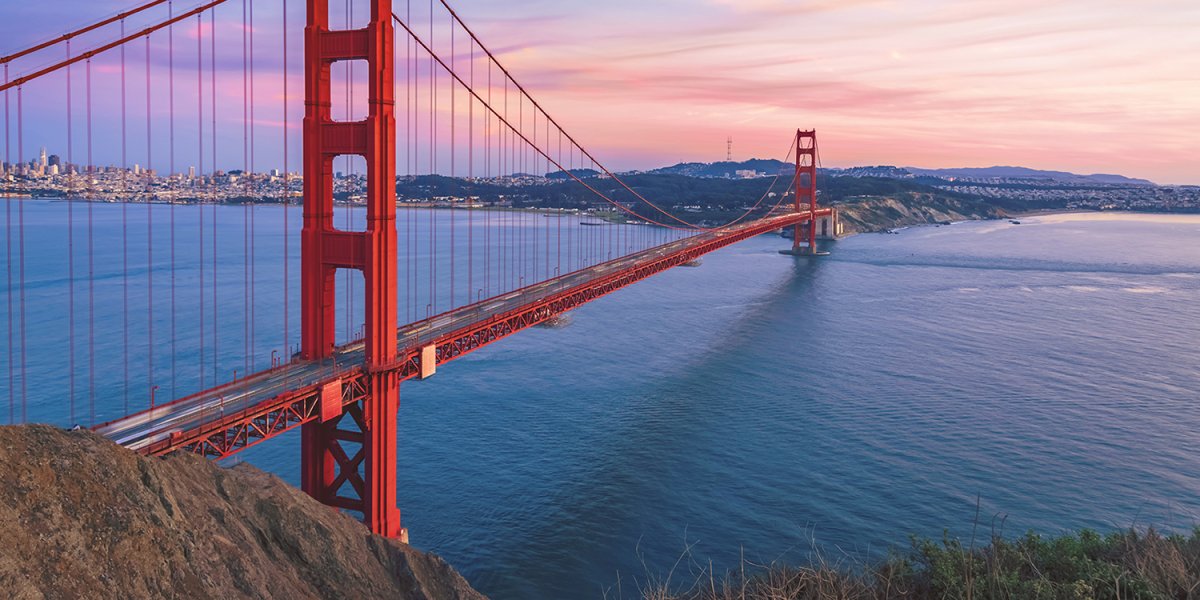This picturesque image captures the iconic Golden Gate Bridge in San Francisco, California, bathed in the serene hues of either a sunrise or sunset. Dominating the scene is the bridge itself, resplendent in its reddish-orange glory and spanning a vast and tranquil ocean, whose still, blue waters stretch out beneath it. The sky above is a beautiful blend of pink, gold, white, and traces of purple, suggesting the transition of day to night or vice versa. In the background, the city's downtown area is visible, with tightly compact buildings, and beyond that, a series of mountains add depth to the landscape. Adding to the natural beauty, there is shrubbery in the foreground, including marshy grass, trees, and a light brown, ragged boulder rock in the lower left corner. Despite some cars zipping past on the bridge, the overall atmosphere is calm and scenic, capturing the beauty and grandiosity of this famous landmark in a moment of tranquility.